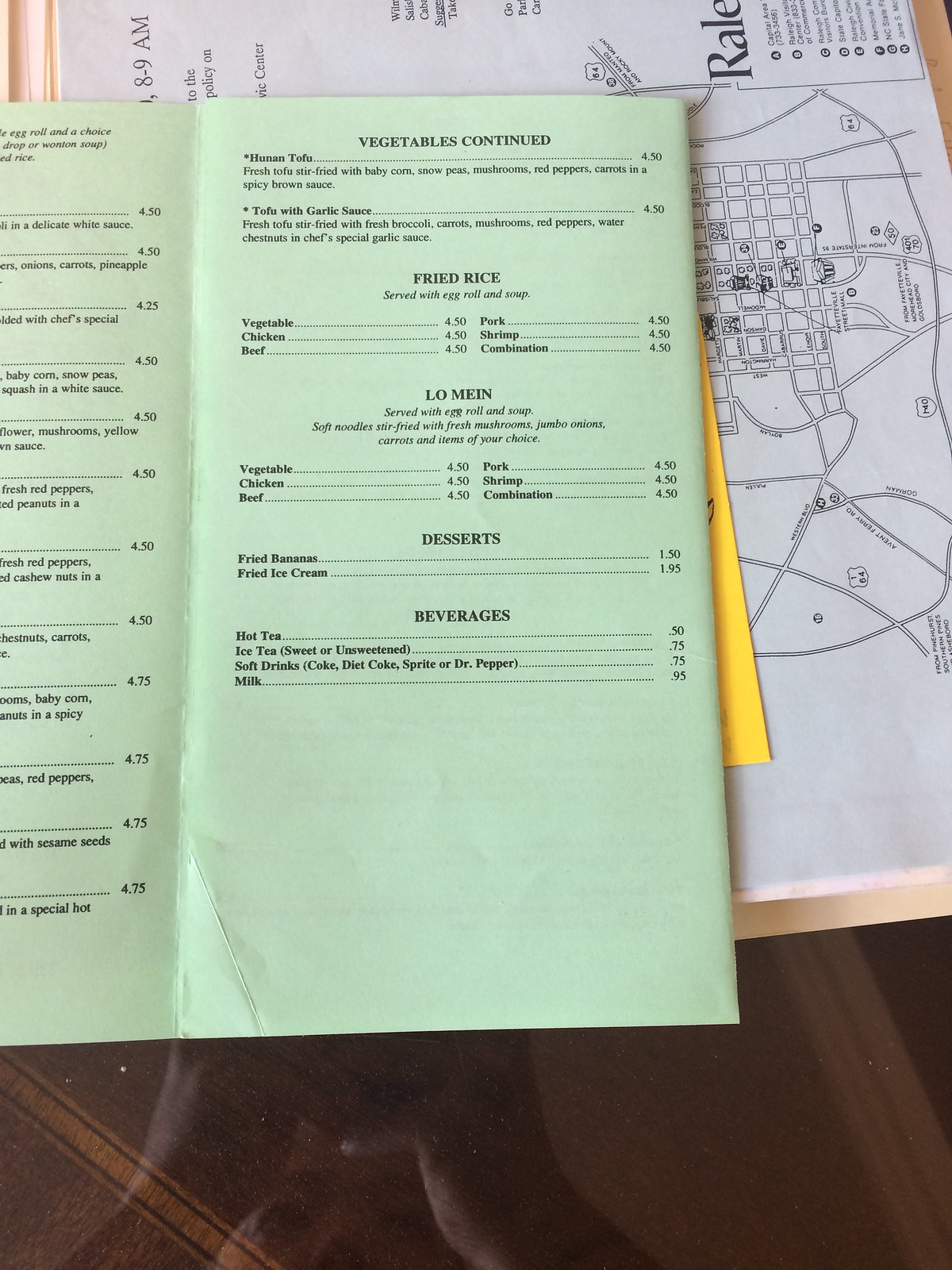In the image, a person is taking a photo of a menu laid out on a table. The menu is opened to two pages, displaying a selection of dishes. The top part of the menu is labeled "Vegetables Continued," listing items such as "Human Toffee" and "Tofu with Garlic Sauce," each priced at $4.50. Further down, bold black text highlights a section for "Fried Rice," with the note "Served with egg roll and soup" detailed just below. This section continues with various combinations of vegetables, chicken, beef, pork, and shrimp dishes. The entire menu is set against a light green background. 

At the very bottom of the image, approximately 10% up from the bottom, there is a faint reflection of the photographer, revealing their white skin tone and partial facial features. In the background behind the menu, there appears to be a map of a city with the word "Rail" visible in the upper right corner. Additionally, a partially visible yellow pamphlet or paper peeks out from underneath the green menu.